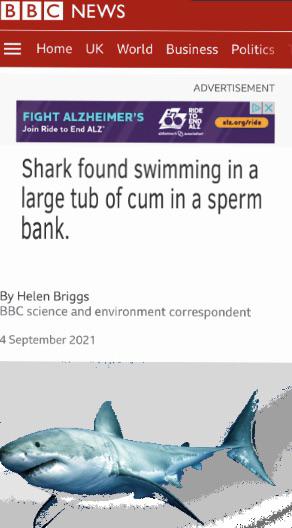This is a detailed description of a screenshot captured from the BBC News app or website. At the top, the iconic BBC News branding is prominently displayed, followed by navigational tabs labeled as Home, UK, World, Business, and Politics. Just below the navigation menu, an advertisement is shown, which reads: "Fight Alzheimer's, Join Ride to End ALZ."

Following the advertisement, the main headline of the article is presented: "Shark Found Swimming in a Large Tub of Cum in a Sperm Bank." The article is authored by Helen Briggs, identified as the BBC Science and Environment Correspondent, and is dated September 4th, 2021. Below the headline, there is a noticeably low-quality image of a great white shark. The image appears somewhat pixelated and is awkwardly cropped, specifically truncating parts of the shark’s fins. The overall screenshot maintains a rectangular shape, offering a glimpse into an unusual and striking BBC News report.